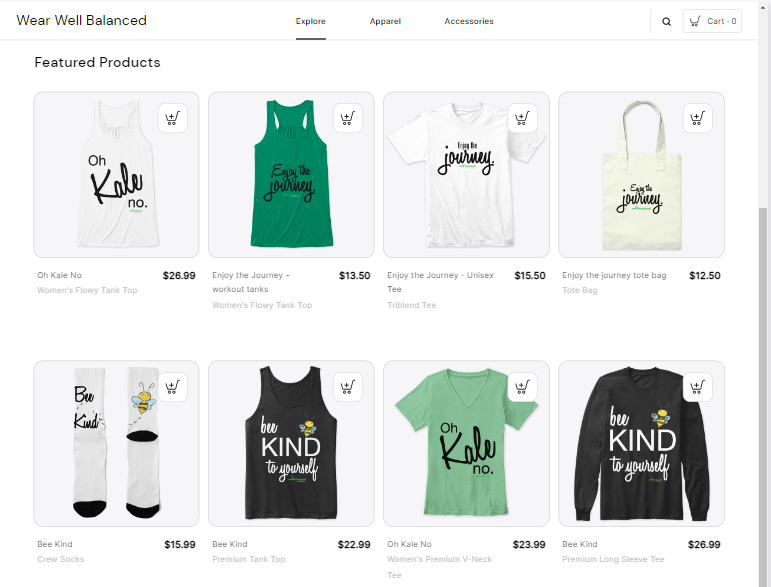In the image, we observe a predominantly white background featuring black text, accompanied by various item images. A gray scrolling bar is visible on the side, which is uncommon for a typical website navigation. At the top, there's a well-balanced arrangement of elements. To the right, a highlighted "Explore" button is present.

The upper section displays categories such as "Apparel" and "Accessory," along with a search icon represented by a magnifying glass, and a cart icon showing a count of 0 items.

Below this, the "Featured Products" section showcases a row of four items, including a variety of apparel. Detailed descriptions and prices of the items are provided:

1. **Oh, Kale No Women's Flowy Tank Top** - priced at $26.99.
2. **Enjoy The Journey Workout Tank** - $13.50.
3. **Enjoy The Journey Unisex Tri-Blend Tee** - $15.50.
4. **Enjoy The Journey Tote Bag** - $12.50.

Additional items are listed beneath the featured row:

5. **Be Kind Crew Socks** - $15.99.
6. **Be Kind Premium Tank Top** - $22.99.
7. **Oh, Kale No Women's Premium V-Neck Tee** - $23.99.
8. **Be Kind Premium Long Sleeve Tee** - $26.99.

The apparel items mainly feature white, green, and black colors.